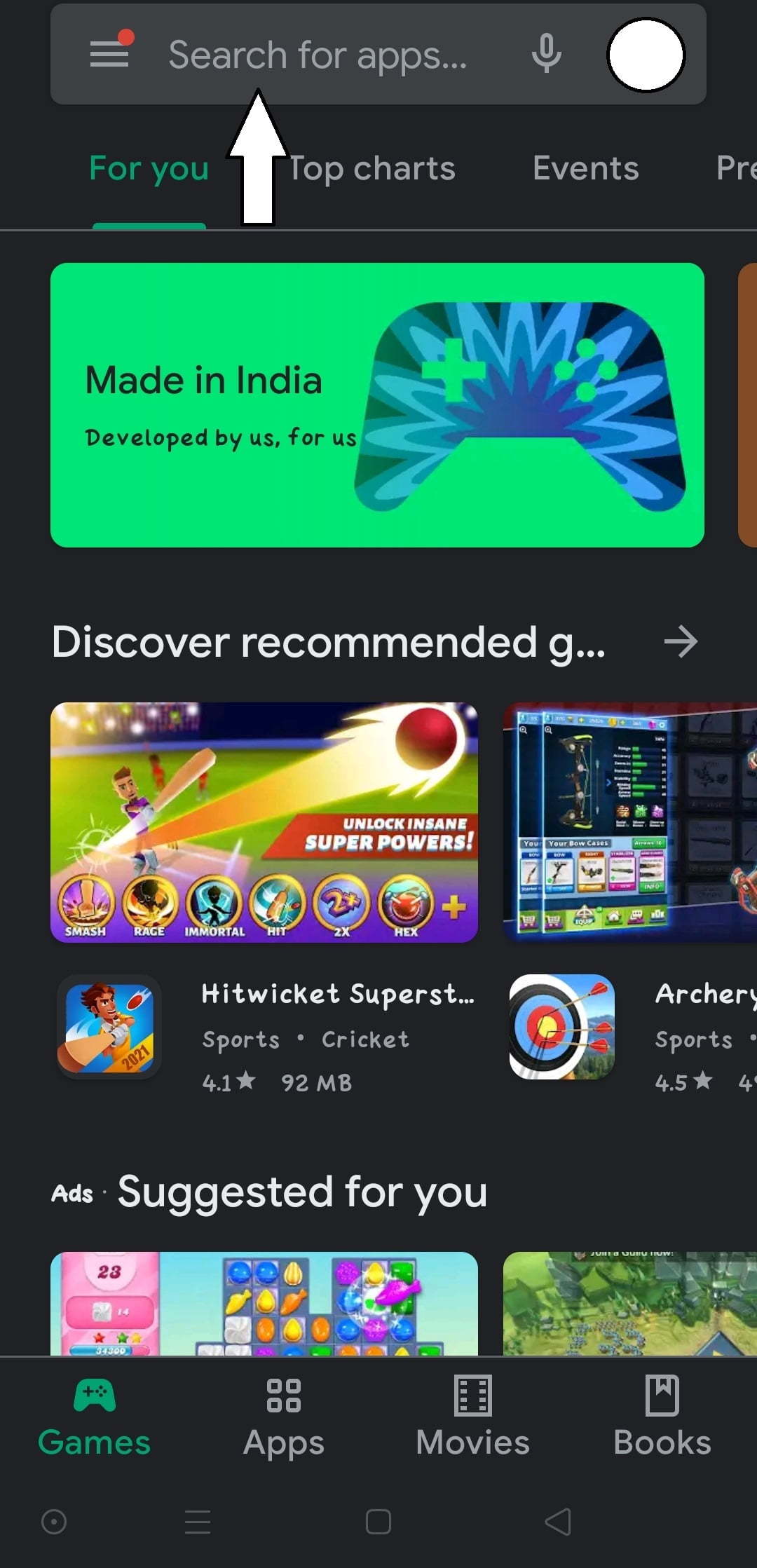The image is a screenshot from a smartphone displaying a dark gray, nearly black background. At the top center, there is a dark gray search box, slightly lighter than the overall background. Within the search box, the text "Search for apps" is visible. To the left of the search box, there are three horizontal gray lines with a dot above them, representing a drop-down menu. On the right side of the search box, there's a microphone icon for voice search, and a white circle is situated at the far right.

Beneath the search box, a large green rectangle stands prominently, featuring the text "Made in India" in black font and the slogan "Developed by us, for us." Adjacent to this text is an image shaped like a game controller with a starburst design in shades of blue. A white arrow points from this rectangle to the search box.

Further down, a white headline reads "Discover recommended G", which likely stands for games. Below this, there is a screenshot of a game titled "Hit Wicket Super ST," showcasing a cartoonish cricket field. 

Near the bottom of the screen, the text "Suggested for you" appears, followed by partial images of several game icons. The footer of the screen lists navigation options from left to right: "Games" in green text, followed by "Apps," "Movies," and "Books" in white font.